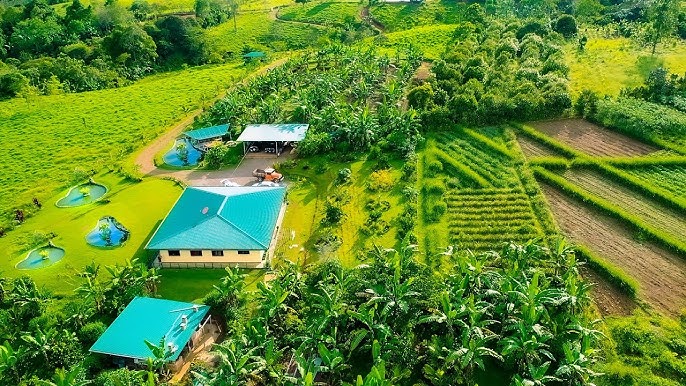This aerial photograph, taken on a sunny day, showcases a lush, vibrant green landscape filled with a variety of plants, predominantly palm trees and farm-like rows of crops. The image features a combination of structures and natural elements, primarily focusing on a set of smaller buildings in the right center. Among these buildings, there are two that resemble smaller homes, each with a bright blue roof—one peaked and the other flat. Flanking them are two additional structures; one with a bright blue roof supported by poles and another with a white roof. Toward the left side of the image, several irregularly shaped ponds filled with bright blue water are visible, adding a striking contrast to the green surroundings. The right side of the image displays a patch of farmland with brown tilled rows of soil, some planted and others not, indicating agricultural activity. The entire scene is suffused with rich, saturated greens and hints of yellow-green, showcasing a lush, almost jungly environment.